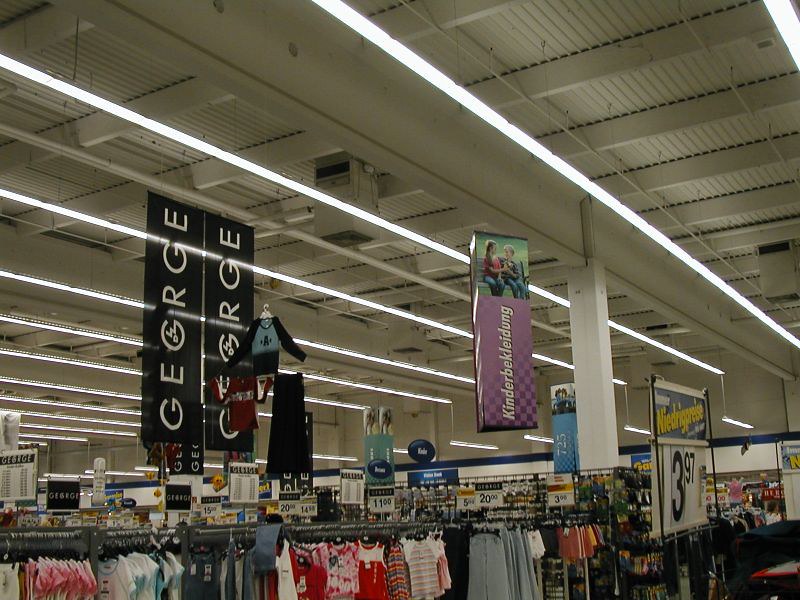The photograph captures the interior of an apparel store, angled upwards toward the white ceiling adorned with several vertical lines and bright rectangular lights, likely fluorescent or LED. Suspended from the ceiling, a heating unit and a series of long bar lights stretch from left to right. Prominently featured are two large, rectangular signs with the brand name "George" emblazoned in white text on a black background, linked to the ceiling rafters. In the foreground, a fixture displays a price sign of $3.57, written in yellow text. The lower half of the image showcases various clothing racks abundant with children's apparel in vivid colors including red, blue, white, and pink. Towards the back, the store's rear wall is visible, accentuated by a blue line that runs along the top. The comprehensive array of details underscores the bustling and vibrant retail ambiance.